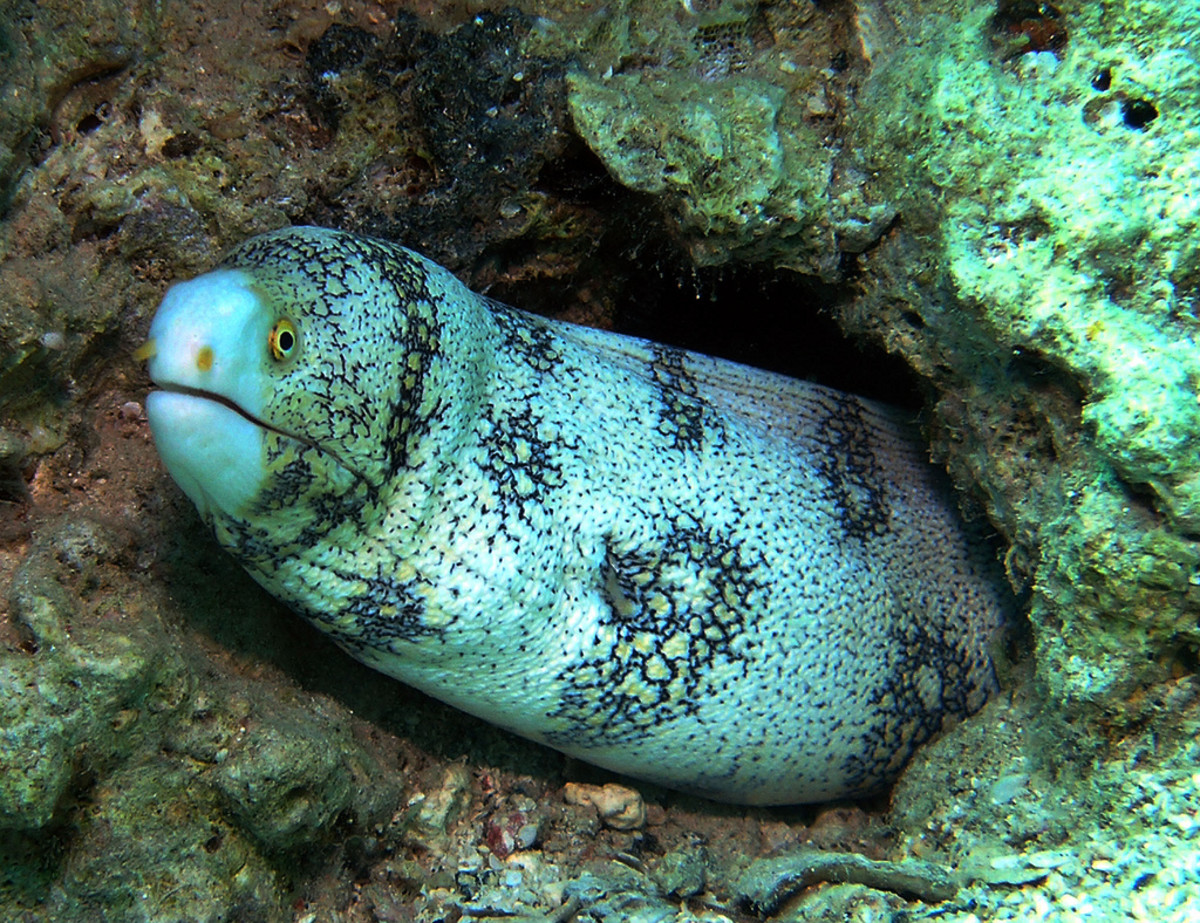This underwater nature photograph captures a striking moray eel peeking out of its hiding hole in a coral reef. The eel has a light blue or bone-white base color, adorned with a random pattern of dark and orange markings scattered across its body, giving it a stained appearance. Its eyes are a vivid yellow, and it possesses two tunnel-like nostrils on its snout. The eel's mouth is notably wide. The reef or rocks surrounding its hiding hole share light blue and green hues, blending harmoniously with the eel's coloration. The image is undoubtedly taken with a waterproof camera, ensuring the eel and its underwater habitat are depicted in detail as the eel emerges, head first and facing forward, from the left side of the composition. The intricate and colorful patterns on the eel's body add to the visual interest of this immersive underwater scene.